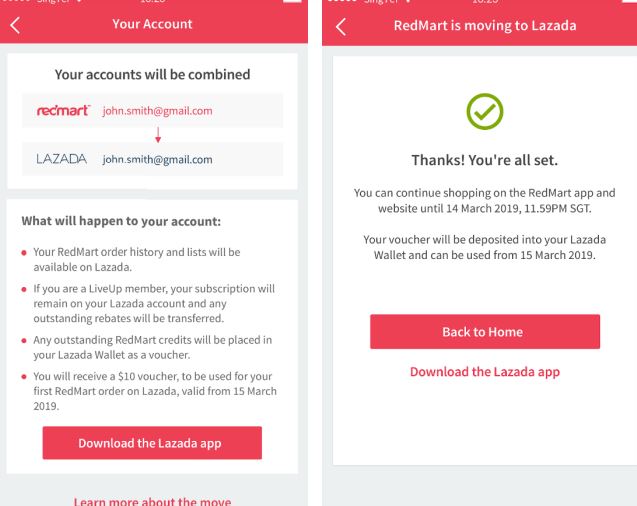The image consists of two screenshots from a mobile device, detailing the integration of RedMart and Lazada accounts. 

The first screenshot provides detailed instructions on the merging process of the two accounts. It includes the user's email address and outlines important information such as the continuity of order history and lists. It ensures LiveUp members that their subscription will remain intact within Lazada and states that any outstanding credits will be combined. The screenshot also features a downloadable button for the Lazada app.

The second screenshot illustrates the completion of this integration. It prominently displays a green arrow enclosed in a circle with a confirmation message, "Thanks, you're all set." It informs users that they can continue shopping on RedMart until March 14, 2019. Additionally, it mentions that a voucher will be deposited in the Lazada wallet, which will be available for use starting March 15, 2019. Below this message, there is a button labeled "Back to Home," along with another link to download the Lazada app.